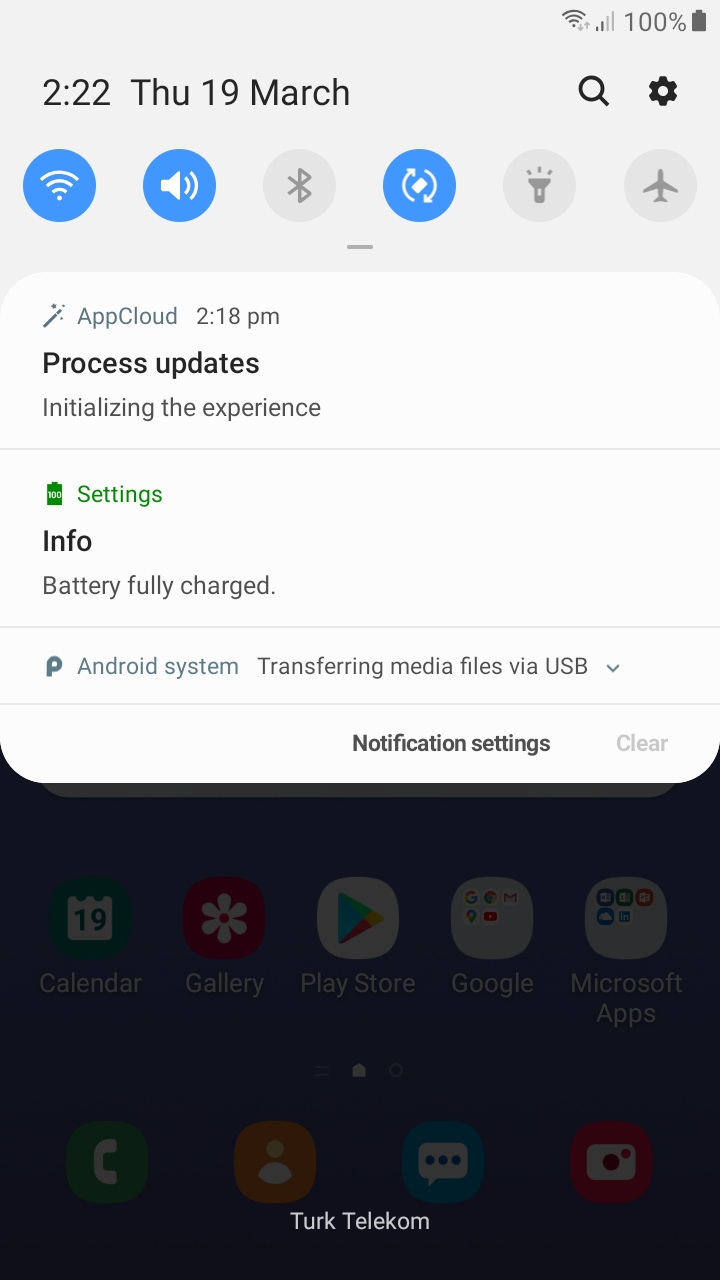The image depicts a screenshot of a cell phone displaying a notification center and settings menu overlay. 

At the top of the screen, there's a light gray status bar. On the right side of this bar, icons indicate a strong Wi-Fi signal, full cellular reception, and a 100% battery charge. 

Below the status bar, on the left side, the date and time are displayed: "2:22 - Thursday, 19 March." On the same line, towards the right, there are icons for "Search" and "Settings."

Underneath this, there's a semi-transparent menu, which appears to be the quick settings panel typically accessed by pulling down from the top of the screen. This panel includes icons for various functions such as Wi-Fi, Sound, Bluetooth, Rotate, Flashlight, and Airplane Mode. The Wi-Fi, Sound, and Rotate icons are highlighted in blue, indicating they are active, while the others remain gray.

Further down, on a white background, notifications are listed. The first notification reads "Apple Cloud 2:18 PM," followed by tasks such as "Process Updates" and "Initialize the Experience" with a progress line indicating the initialization process.

Additional lines of text include "Settings" highlighted in green, followed by "Info" and "Battery Fully Charged." 

Further down, there is an "Android System" notification detailing actions such as "Referring Media Files," "Use USB," and "Transferring Media Files via USB."

On the lower right corner of this overlay, there are options for "Notification Settings" and "Clear."

This entire notification and settings overlay is displayed over the main screen content.